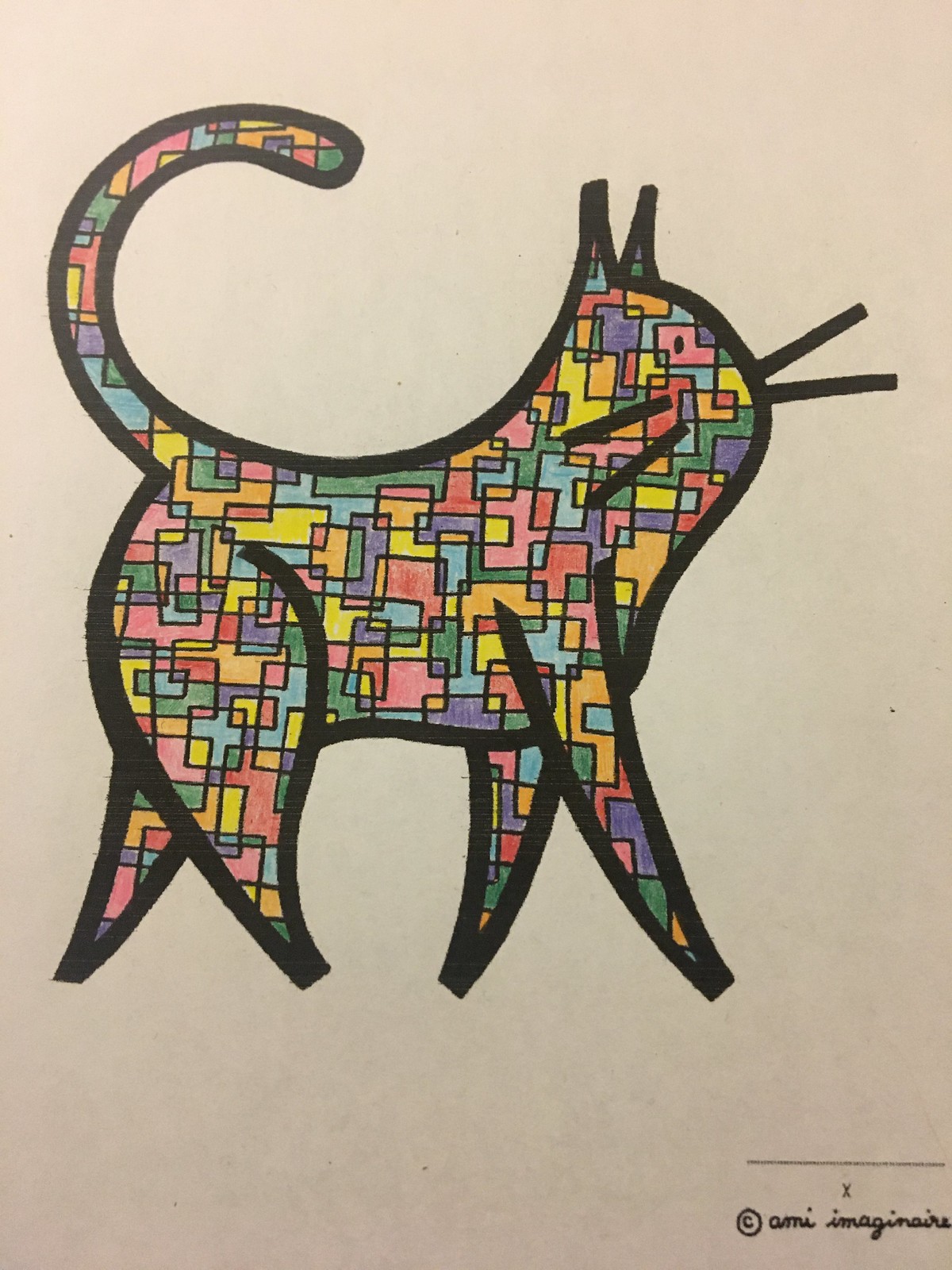A vibrant, cartoon-style drawing of a cat adorns a piece of white paper in this photograph. The cat, captured in a side profile with its head facing the right, is an eye-catching spectacle of geometric artistry. Instead of traditional fur, the cat's body is covered with colorful geometric shapes, predominantly rectangles and squares, splashed with an array of hues including red, purple, yellow, orange, green, and blue. The cat’s tail curves gracefully above its back, forming a C shape. Its pointed ears stand erect, adding a touch of alertness to its character. Solid black whiskers, four in total, jut out symmetrically from both sides of its face. The whimsical cat stands on triangular feet, which lack defined paws, emphasizing its cartoonish design. Encasing the entire figure is a bold black outline, creating a sharp contrast against the white background. At the bottom right corner of the paper, the artist's signature is penned in black, accompanied by a circled letter C and an enigmatic X above a horizontal black line, serving as distinctive marks of the creator's identity.